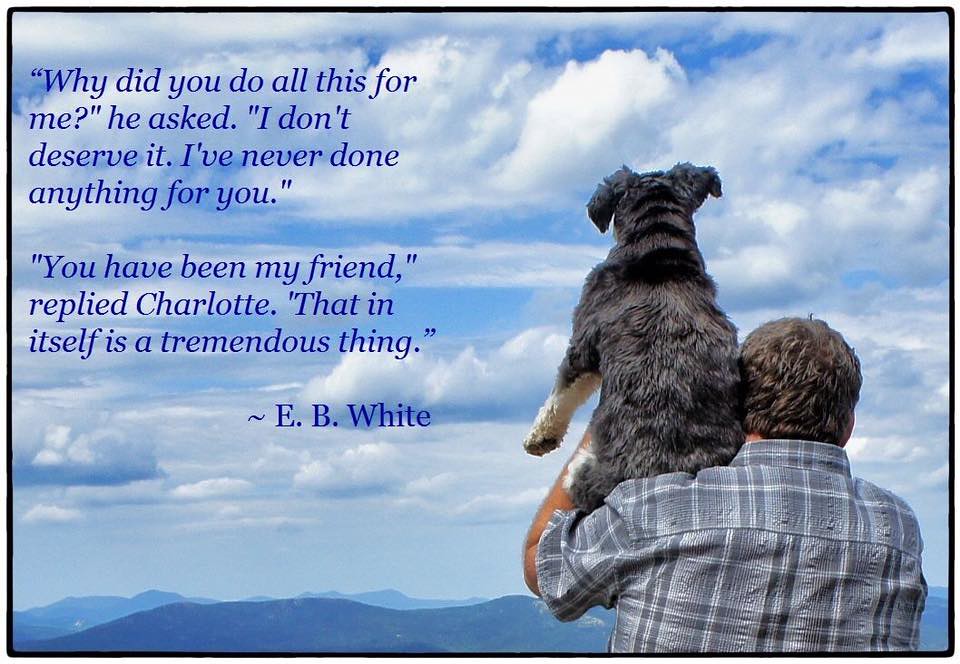In this rectangular landscape image, resembling a picturesque postcard, the background features a serene blue sky adorned with puffy white clouds, gradually transitioning to reveal distant, hazy hills in subtle blue hues and darker low hills beneath. Dominating the bottom right of the image, a man dressed in a short-sleeved, collared button-down shirt with an irregular pattern of black and white stripes stands with his back to the viewer. His dark brown hair brushes his left shoulder as he supports a silvery-dark gray dog, which mirrors the hue of his hair. The dog, perched on his left hand with its white left paw visible, gazes out toward the horizon alongside the man, both facing away from the camera.

Above this tranquil scene, starting in the upper left corner, an eloquent quote from E.B. White's "Charlotte's Web" is presented in dark blue, italicized font: “Why did you do all this for me? He asked. I don't deserve it. I've never done anything for you. You have been my friend, replied Charlotte. That in itself is a tremendous thing.” The quote spans two paragraphs and is clearly attributed to E.B. White beneath it, blending seamlessly with the ethereal, possibly illustrated backdrop that could either be a photograph or a detailed drawing, emphasizing the profound connection between friendship and selflessness against a soothing natural landscape.